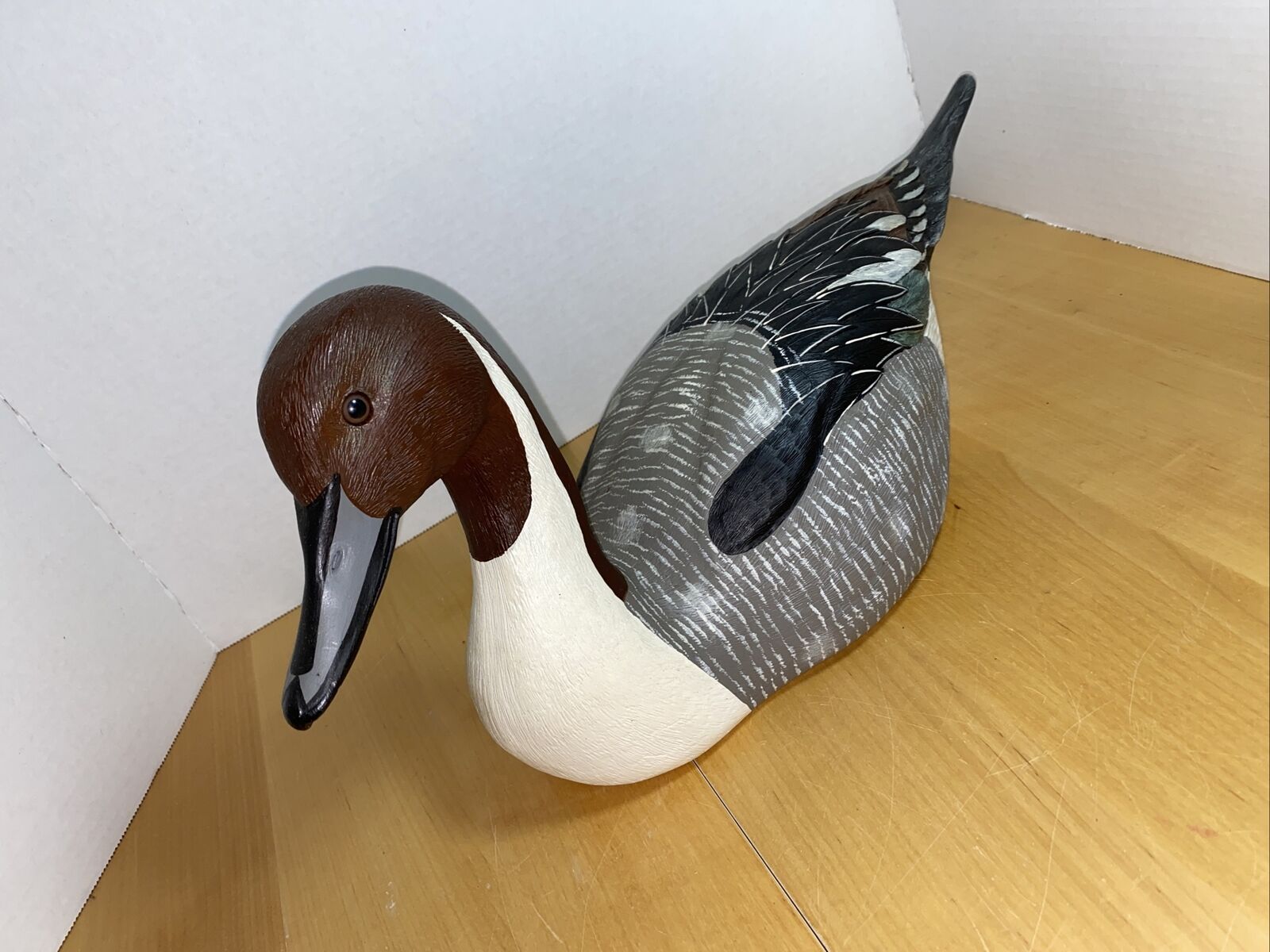This photograph portrays a meticulously crafted wooden duck statue, resting on a light brown hardwood floor in front of a white wall. The duck features a brown head with a glossy black bill that has silver stripes on either side, and it possesses a notably realistic appearance despite its wooden material. The bird's eye is a deep brown and glossy. Starting from the neck, the feathers transition to a vivid white that extends down to its silvery-gray body adorned with white stripes. The sides and back of the duck are marked with more elaborate, darker patterns: triangular black feathers, a transitional black cylindrical shape, and finally, a dark bluish tail with intricate white and gray feather outlines. The statue casts a subtle shadow above its head, hinting at the light source illuminating the scene.